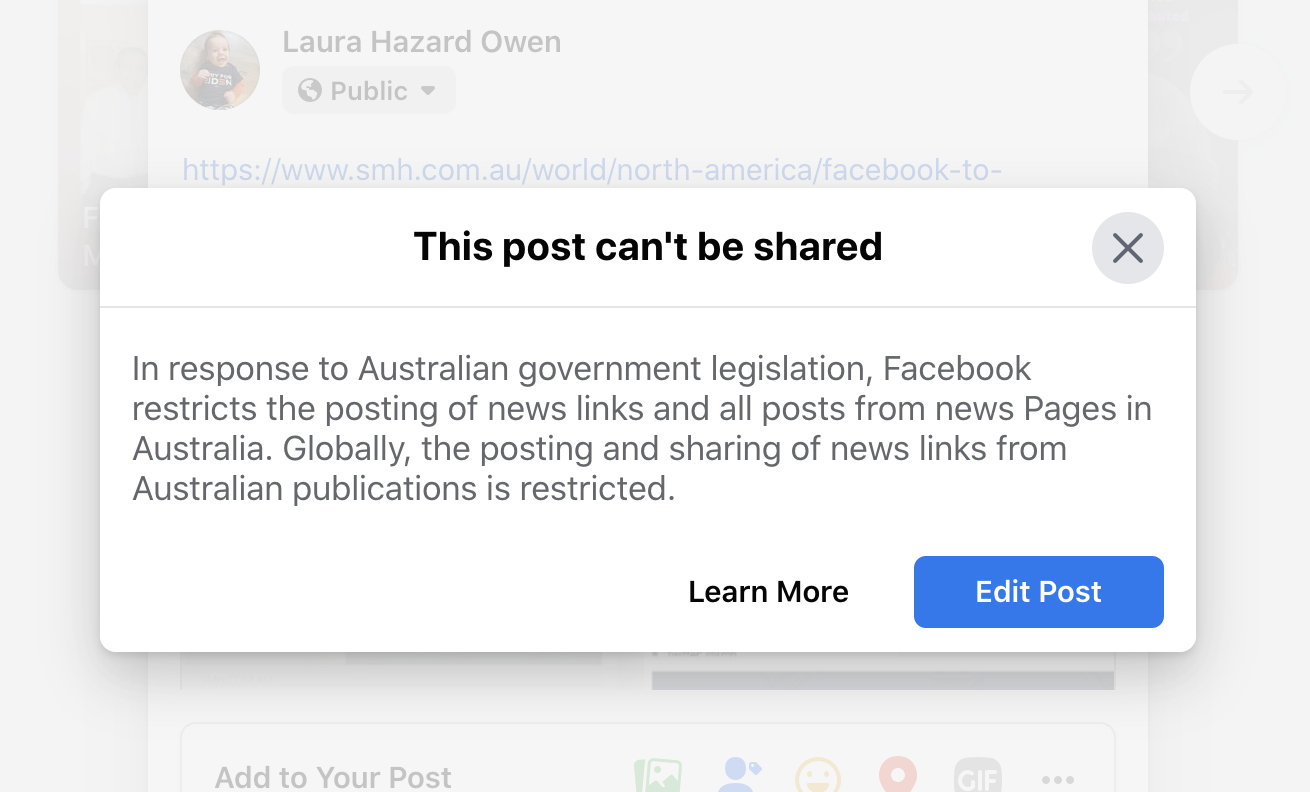The image features a centered pop-up window with a white background. In the backdrop, there is a profile post by Laura Hazard Owen, which includes a profile picture on the left of a baby. Visible elements of the post include the word "Public" with a dropdown arrow and the web address "www.smh.com.au/world/north-america/facebook-to-". 

The pop-up window itself is prominently displayed in the center of the image. At the top center of this window, the text reads, "This post can't be shared." Beneath this, it explains, "In response to Australian government legislation, Facebook restricts the posting of news links in all posts from news pages in Australia." At the bottom right of the window, there is an option labeled "Edited Post."